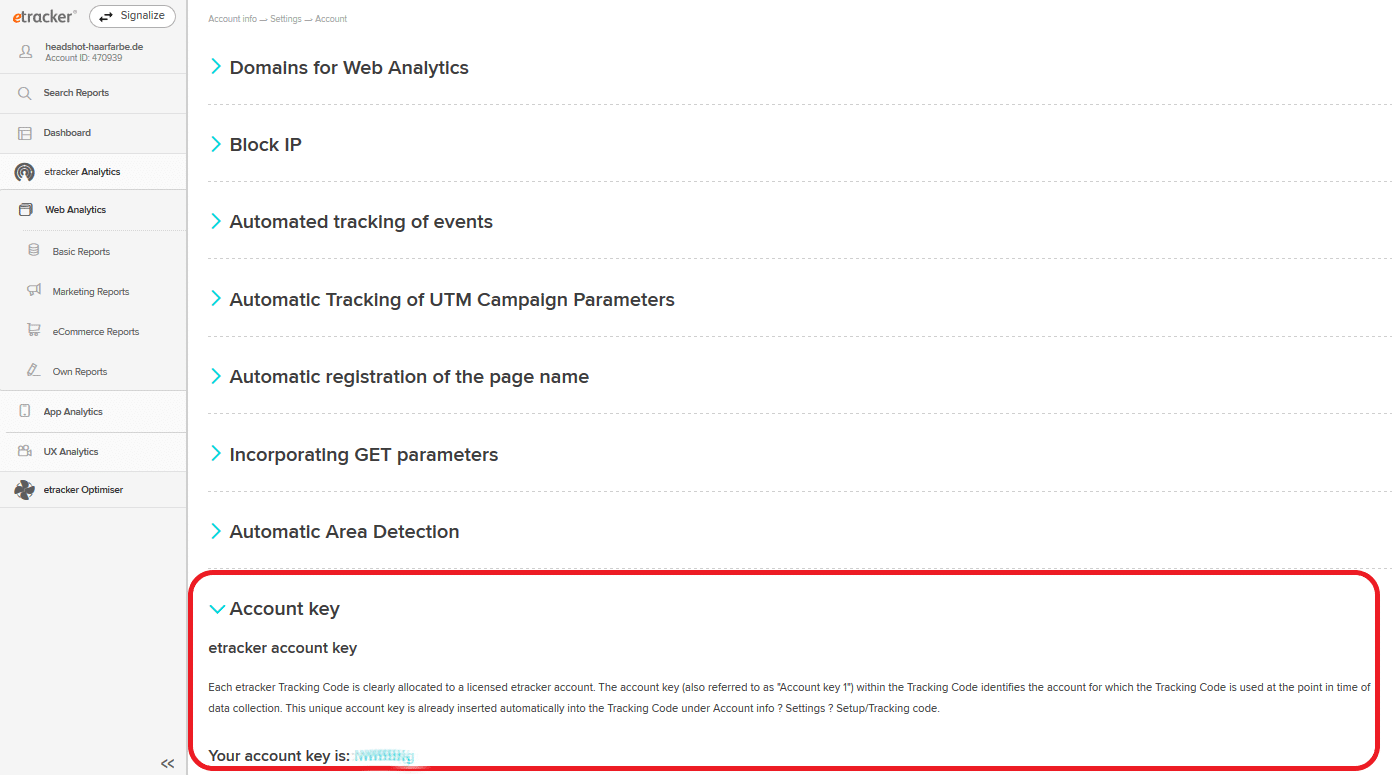The image displays an interface of an e-tracker tool, organized into two primary columns. The first column, shaded in gray, includes a navigational menu with options such as Search Reports, Dashboard, e-Tracker, Analytics, Web Analysis, Basic Reports, Marketing Reports, E-commerce Reports, Own Reports, App Analytics, UK Analytics, and e-Tracker Optimizer. Each of these options presumably expands to reveal further functionalities.

To the right, the second column contains settings related to web analytics and event tracking. This column lists options like Domain for Web Analytics, Block IP, Automated Tracking of Events, Automated Tracking of UTM Campaign Parameters, Automatic Registration of the Page Name, Incorporating Get Parameters, and Automatic Area Detection.

Below these options, there is a prominent white rectangular box outlined in red for emphasis. This box is labeled "Account Key, e-tracker Account Key" and features a description followed by the text "Your account key is:". The actual account key has been redacted for privacy.